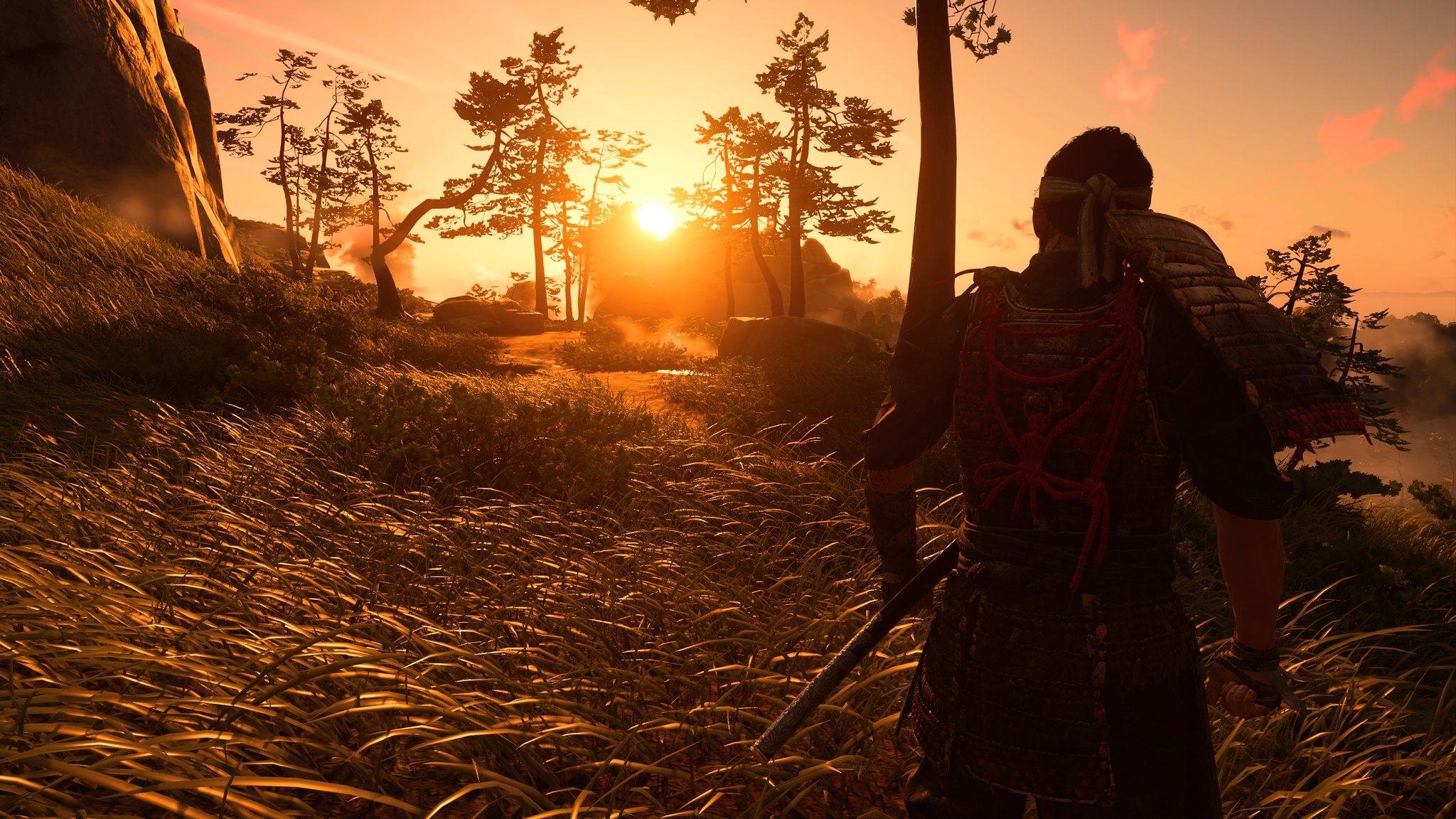In this stunning painting, we observe the solitary figure of a warrior walking through a serene natural landscape. The warrior is depicted from the back, adorned in a black tunic featuring a striking red spider design on the back, and a leather skirt around his waist. Beneath the tunic, he wears a long black shirt, adding layers to his ensemble. A cloth is tied around his head, with the knot resting at the back, and his right wrist is wrapped in leather. He clutches an unidentified object in his hand, partially obscured by his body. On his left forearm, he sports a glove that extends up to his elbow, though it could be a tattoo, adding to his mysterious aura. He carries a long pole, partially concealed from view.

The setting sun casts a warm glow across the scene, its light filtering through tall grasses and distant fog, creating a tranquil yet evocative atmosphere. The horizon is marked by a dense line of trees, behind which the sun is setting. To the left of the composition, a large rocky cliff rises, adding a rugged touch to the landscape. The warrior strides through the grassy expanse, his path suffused with nature’s quiet beauty, lending a contemplative mood to this evocative artwork.